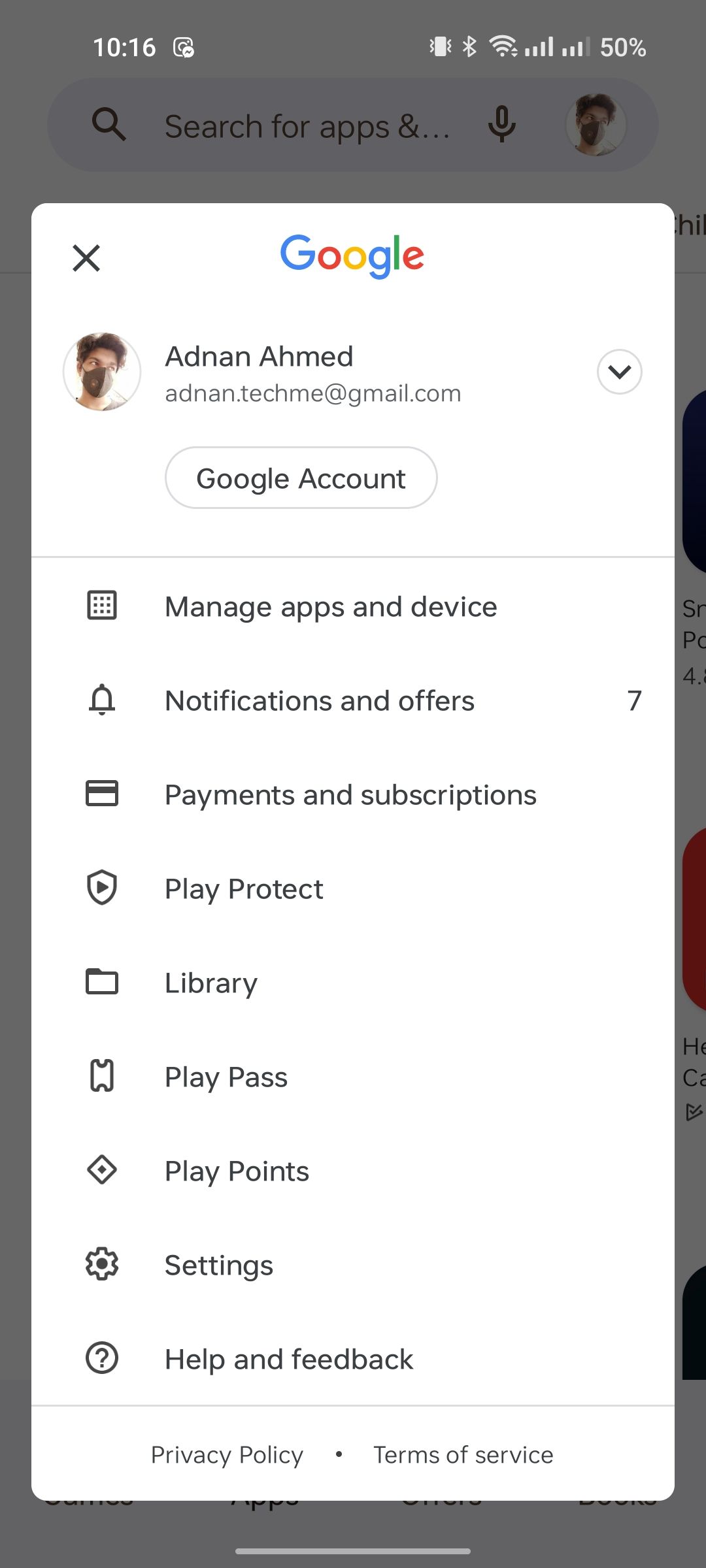The image in question is a screengrab of a mobile phone, formatted in a landscape orientation that's approximately three times wider than it is tall. At the center of this image is a dominant window occupying around 80% of the screen space, leaving the background elements grayed out and less prominent. 

This main window features a stark white background and is bordered in a way that leaves approximately 20% of the space at the top and 10% at the bottom uncovered. In the top-left corner of this window, a small 'X' icon is visible, indicative of a close function. Centrally positioned at the very top is the recognizable Google logo. 

Below this branding element resides a profile section. A man wearing a COVID-19 mask occupies the profile picture space. To the right of this image, the name "ADNAN Ahmed" is displayed prominently, followed by an email address, "ADNAN.techme@gmail.com." 

Further down the window is a clearly defined button with a gray outline and white fill, containing the black text "Google account." 

Below this button, a horizontal gray line separates the profile section from a list of nine different navigational icons, each accompanied by descriptive black text. These icons and their associated functions read as follows: 
1. Manage apps and device
2. Notifications and offers
3. Payments and subscriptions
4. Play Protect
5. Library
6. Play Pass
7. Play Points
8. Settings
9. Help and feedback